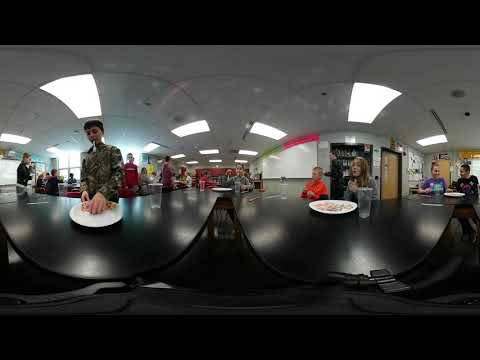The image captured appears to be taken from spy cam glasses, depicting a bustling indoor school lunchroom filled with adolescent children. The scene is somewhat blurry, showcasing a variety of activities and interactions among the students. Some kids are seated at black tables, eating from white trays and plates, with clear plastic cups and glasses with straws scattered around. One notable child on the left, who is wearing a black coat, is seen holding a white food utensil in his mouth while picking up food, possibly from a piece of pepperoni pizza on a white plate. Another child in an army-patterned shirt is engaged in a similar activity. 

In the background, a blend of standing and seated students in dark clothing are visible, with a few engaged in conversation. Notable mentions include a child in an orange shirt sitting next to someone in a gray shirt, and other kids in black and purple shirts seen talking to each other. A vending machine is discernible in the back, adding to the typical lunchroom ambiance. The environment is well-lit with white fluorescent lights, and the walls adorned with various colors like pink, green, and yellow, along with some unreadable signs. Red and white doors frame the active lunchroom setting, reinforcing the school environment where the children are gathered, suggesting they're taking a break to enjoy their meals.